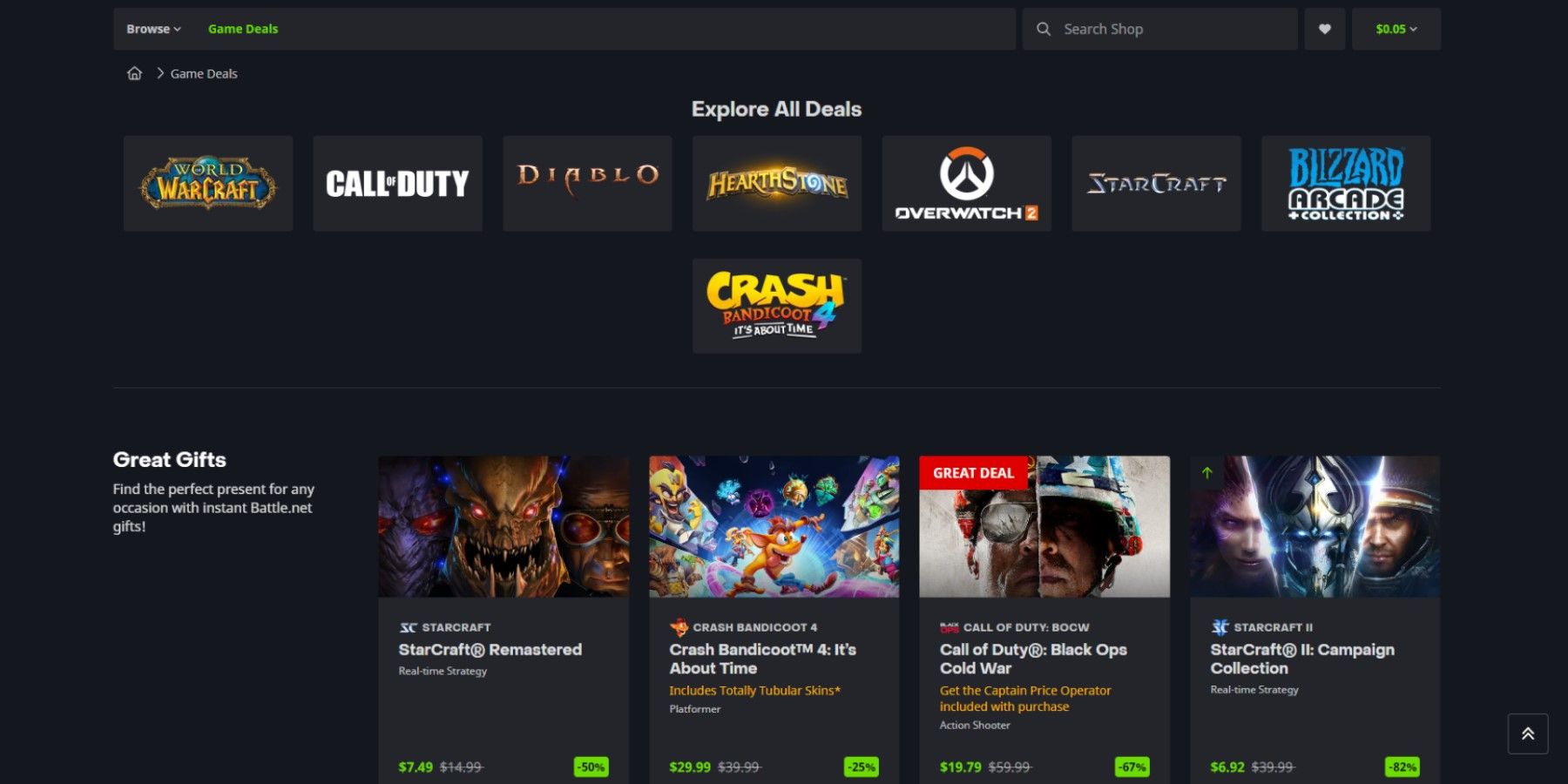Certainly! Here’s the cleaned-up and detailed caption:

---

The screenshot features a user interface with a predominantly black background. At the top, there is a dark gray horizontal banner. On the left side of this banner, it contains the word "Browse" in gray, accompanied by a downward-pointing arrow resembling a lowercase 'v'. To the right of "Browse," the word "Search details" appears in green text. Further right, there's a search box with a gray magnifying glass icon on the left, labeled "Search shop."

Continuing to the right, there is a solid square icon with a white heart inside, and adjacent to it is a box displaying a green dollar amount accompanied by a downward-pointing gray arrow.

Below the top banner, on the left side, there is a house icon followed by a right-pointing gray arrow and the text "Game Deals." Centered two lines beneath this, the white text reads "Explore All Deals." Under this, horizontally-aligned rectangular buttons list popular game titles: Warcraft, Call of Duty, Diablo, Hearthstone, Overwatch, Starcraft, Blizzard Arcade, and a final one for Crash under the Hearthstone section. 

A thin, light-gray horizontal line separates these elements. Approximately three lines below this, in white text, it reads "Great gifts." Below that is smaller white text stating, "Find the perfect present for any occasion," followed by text too small to discern.

On the right side of this section, there are four squares, each containing an image at the top, descriptive text of what it is in the middle, and a lime green square with black writing in the bottom right corner of each.